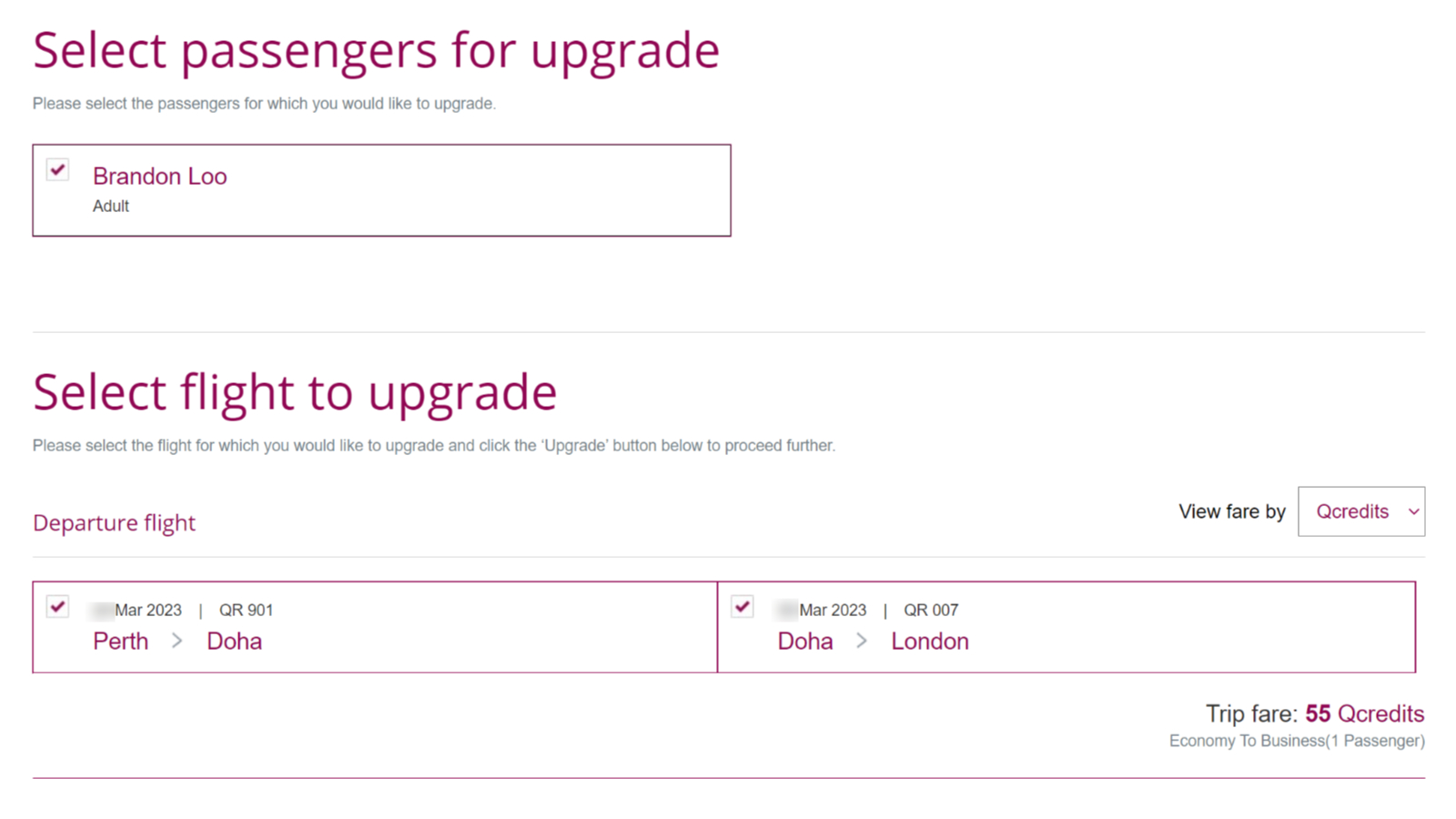The image frame, horizontally rectangular in shape, is a screen grab of a partial webpage dedicated to upgrading passengers on a flight. At the top left corner, there is a prominent purple section titled "Select Passengers for Upgrade." Directly below this heading, there is a smaller, gray font instruction: "Please select the passengers for which you would like to upgrade." Underneath this, there is a horizontal rectangle outlined in purple, containing a checkmark in the top left corner followed by the name "Brandon Liu" in purple text. Below the name, the label "Adult" appears in gray font.

The next section, indicated with large bold text, is titled "Select Flight to Upgrade." Accompanying this heading, smaller gray text provides guidance: "Please select the flight for which you would like to upgrade, and click the upgrade button below to proceed further." Underneath this instruction, the label "Departure Flight" appears in purple on the left side, while "View Fare By" with a drop-down menu box is located on the right side of the screen.

Beneath the "Departure Flight" section, there are two horizontal rectangles side by side, both outlined in purple. These rectangles represent two different flights selected for upgrade: one is for "March 2023, Perth to Doha" on the left, and the other is for "March 2023, Doha to London" on the right. Finally, on the lower right side of the image, the trip's fare is listed as "55 Q Credits, Economy to Business, one passenger."